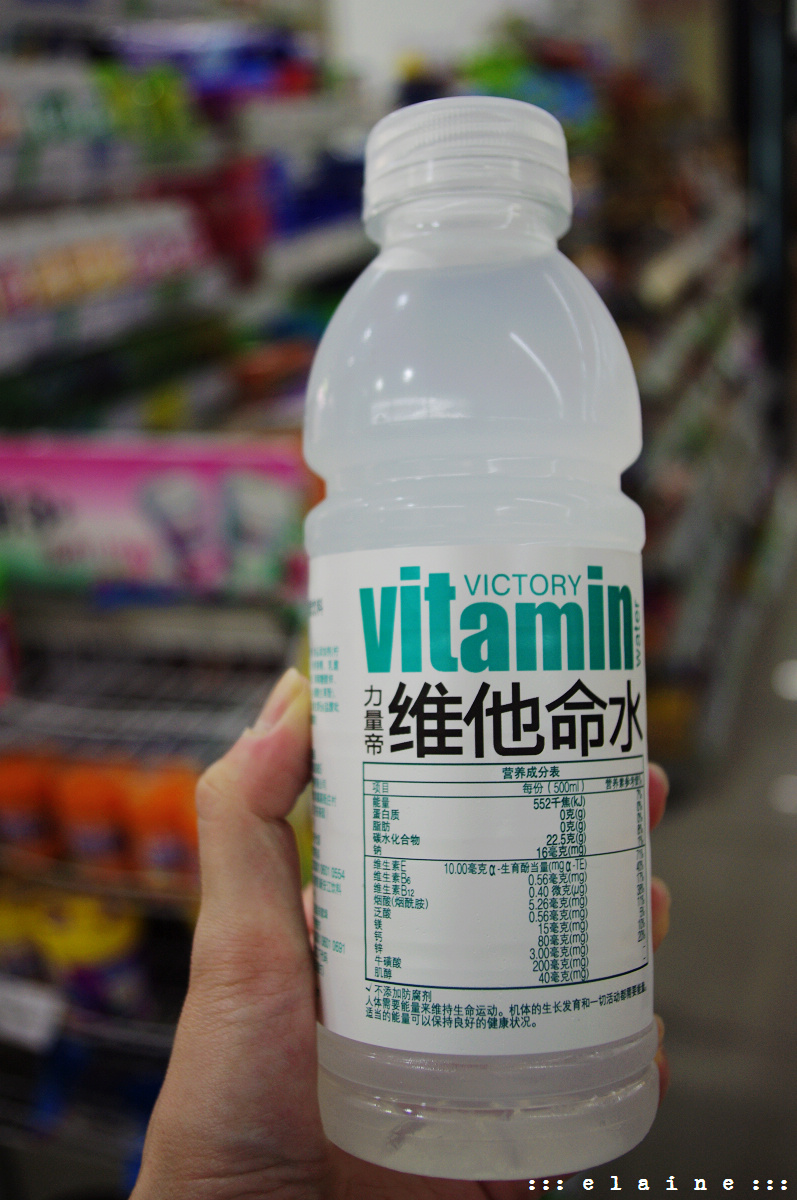In this close-up photograph, a woman's hand enters the frame from the left side, delicately holding a bottle of a white-colored beverage. The bottle itself is transparent with a clear cap, allowing a full view of its contents. The label on the bottle is predominantly white adorned with black and teal text in a foreign script, likely Chinese. At the top of the label, the word "Victory" is prominently displayed, followed by the word "Vitamin" underneath. The detailed nutritional information, also in the foreign script, is visible on the bottle, characterized by distinct symbols. The background of the image is intentionally blurred, yet discernible enough to suggest a setting such as a convenience store or gas station, with displays of candy, chips, and other beverages faintly visible. In the bottom right corner of the image, the name "Elaine" is subtly printed in white lettering, adding a personal touch to the scene.